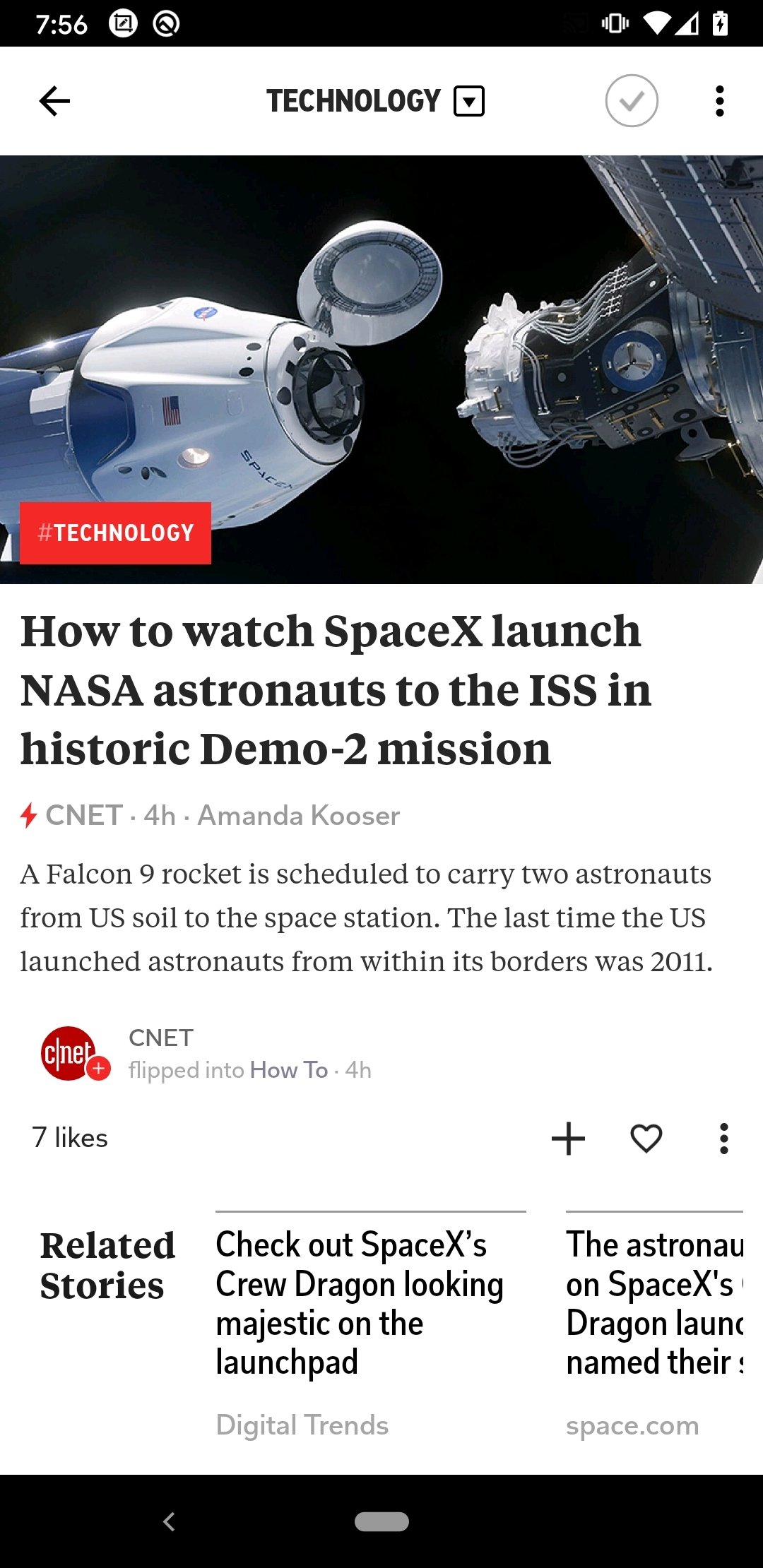This image is a screenshot of a technology-related webpage. At the top, it features a drop-down menu within a square that includes a left-pointing arrow and a check mark, both in grey, as well as a three-dot menu in the upper right-hand corner.

The main visual element of the image is a photograph of a SpaceX spacecraft preparing to dock with the International Space Station (ISS). The spacecraft is distinguished by its white cone-shaped top that has been lifted, revealing a blue main body. 

In the bottom left corner of the picture, there’s a red box with the word "Technology" written in white. Below this box, text reads: "How to watch SpaceX launch NASA astronauts to the ISS in historic Demo-2 mission." Accompanying this is a red lightning bolt icon next to the text "cnet.4h.amandacusa." Additional text explains that a Falcon 9 rocket is scheduled to carry two astronauts from U.S. soil to the space station, marking the first U.S.-based astronaut launch since 2011.

Below this, there's a maroon circle with "CNET" written inside it and a red circle with a plus sign. Grey text adjacent to these icons reads "CNET," followed by "howto.4h." The caption indicates the post has received seven likes, shown in black text. To the right, there are icons for a plus sign, a favorite tag, and another three-dot menu.

Underneath the main text, a section titled "Related Stories" is displayed. The first related article, separated by a short grey line, invites users to "Check out SpaceX's Crew Dragon looking majestic on the launch pad," credited to Digital Trends in grey text. Another partially visible article underneath mentions "The astronaut on SpaceX's dragon launch," credited to Space.com in grey text.

The bottom of the image features a black bar containing a grey left arrow and a grey oval in the center.